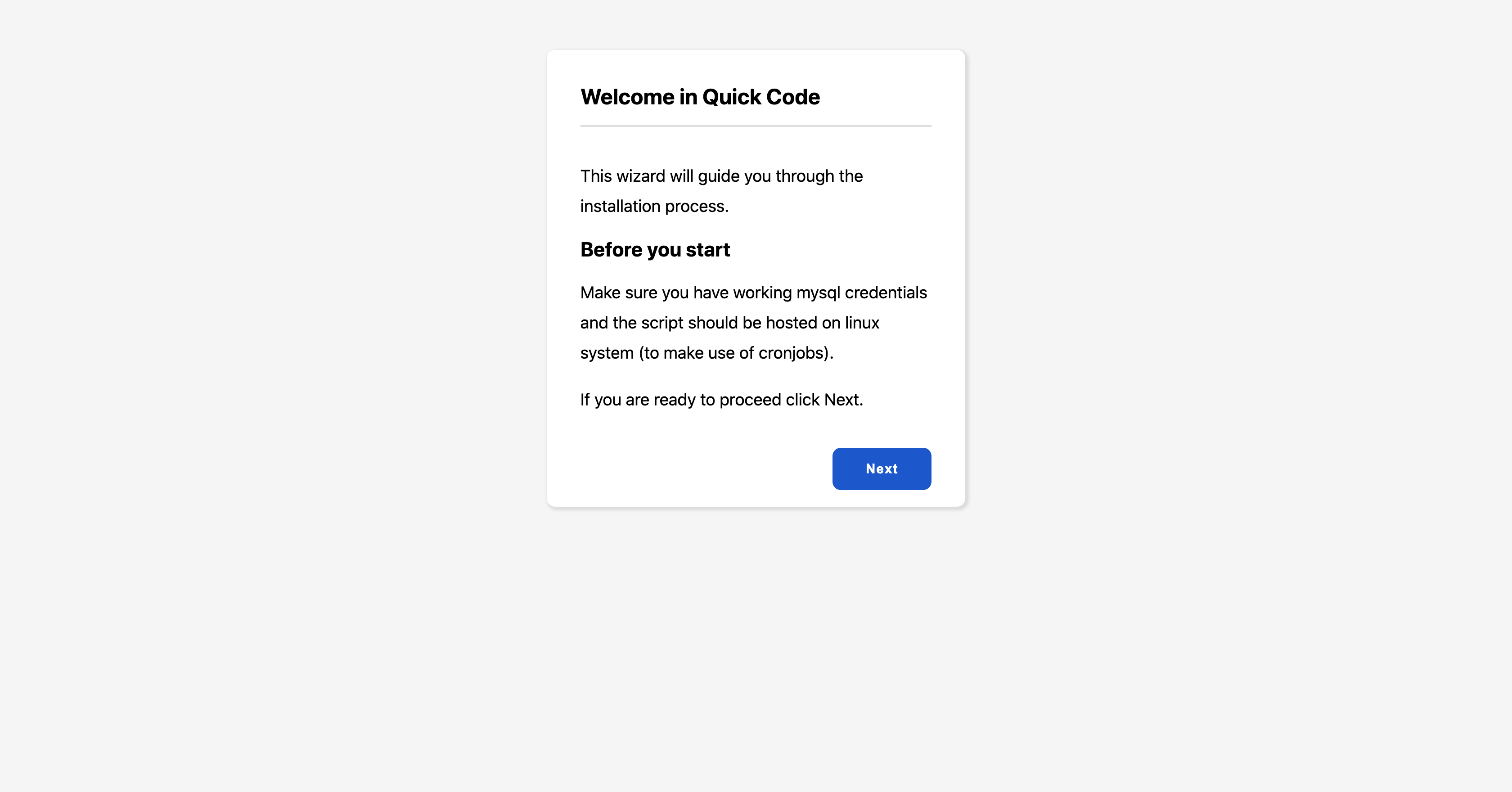Detailed Descriptive Caption:

"An image showing a pop-up message on a computer screen. The pop-up has a clean, simple design with a white background and black text. The heading reads 'Welcome to QuickCode.' Below the heading, the message introduces a wizard that will guide the user through the installation process. It advises ensuring that the user has working MySQL credentials and that the script is hosted on a Linux system to utilize cron jobs. At the bottom of the pop-up, there is a prominent blue button labeled 'Next,' inviting the user to proceed with the installation."